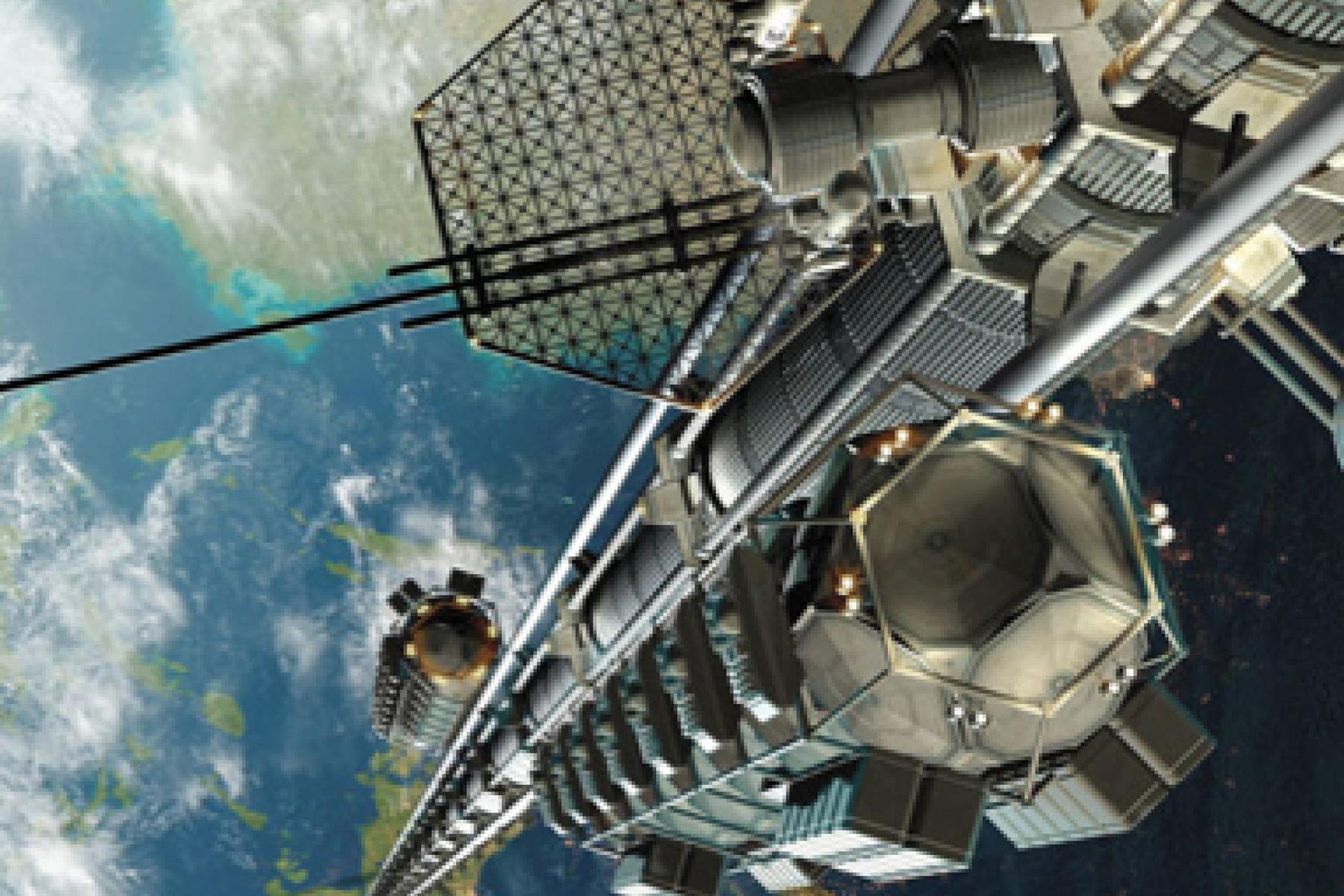The image is a highly detailed, full-color, computer-animated piece, portraying an artistic interpretation of a spacecraft in space, illuminated by natural light. The square composition prominently features the Earth on the left half, showcasing swirling white clouds, expansive blue oceans, and distinct brown and green land masses beneath a thin veil of clouds. The right side and lower portion of the image fades into the inky blackness of space. 

Dominating the foreground is a long, segmented space station, partially captured in the frame, suggesting that the camera is mounted on one end of the structure. The spacecraft exhibits a variety of intricate mechanical components including rectangular metal segments, thin metallic materials, and a very long antenna or transmission tower extending to the left. The space station's primary color is a utilitarian gray, highlighting its industrial design devoid of any visible weaponry. The image intricately details the complexities of the spacecraft's interconnected parts, such as propulsion systems, engines, and circuitry, set against the stunning backdrop of our planet far below.